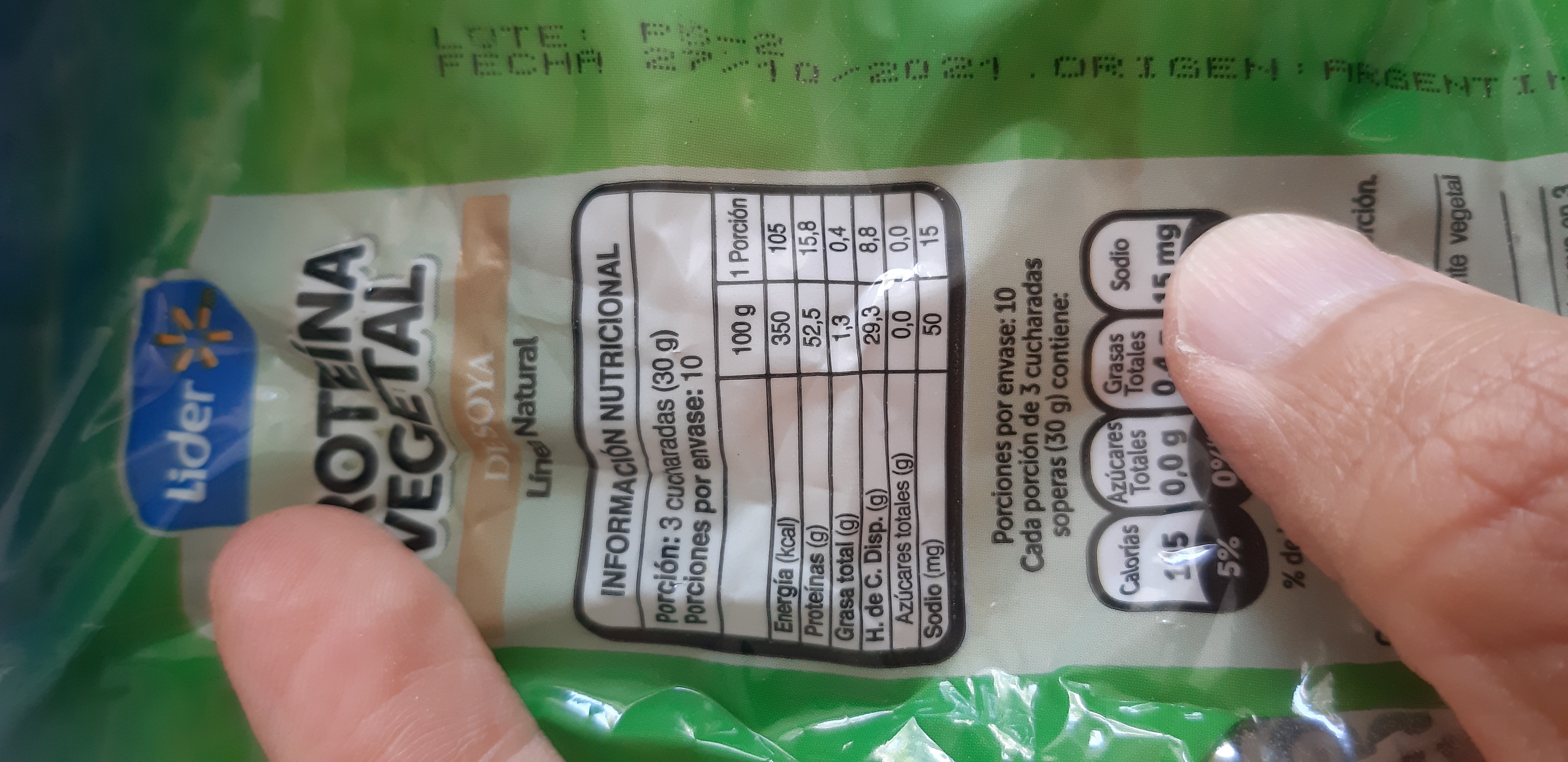A close-up photograph showcases a partly obstructed food package being held between two fingers against a light brown background. The package, titled "LIDER" in white letters on a blue background with a yellow-orange flower emblem, is primarily green with a horizontal silver strip displaying nutritional information and ingredients in Spanish. The package is oriented sideways, causing the details to be listed from left to right, with a finger blocking part of the sodium information. Large text reading "Proteína Vegetal" followed by "DISOYA" in a white banner, and "Lying Natural" in black are prominently displayed. The top mentions "LOTE PS-2" and "Fecha 27/10/2021" as well as "Origen: ARG..." with the full country of origin obscured. Nutritional info includes details like calories and percentage values, framed by small white and black ovals.